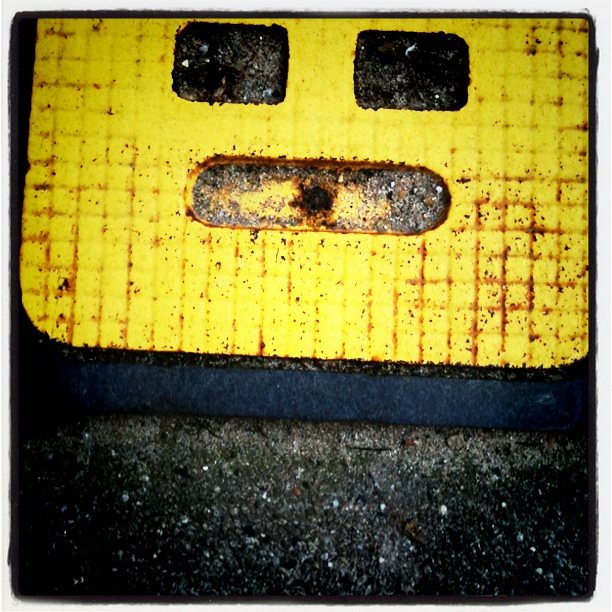The image depicts a rectangular, yellow, metal object, heavily rusted and worn, situated on a black asphalt surface sprinkled with white specks, which appears to be a road. The yellow object has a grid-like pattern with multiple rust spots and indented areas adding to its textured appearance. Its overall shape is rectangular with rounded edges, and notable features include two rectangular cutouts near the top, resembling eyes, and an oval-shaped area in the middle, which could be interpreted as a mouth or a grimace, giving it a face-like appearance. The contrast between the bright yellow, rust, and black asphalt highlights the stark visual and textural differences.